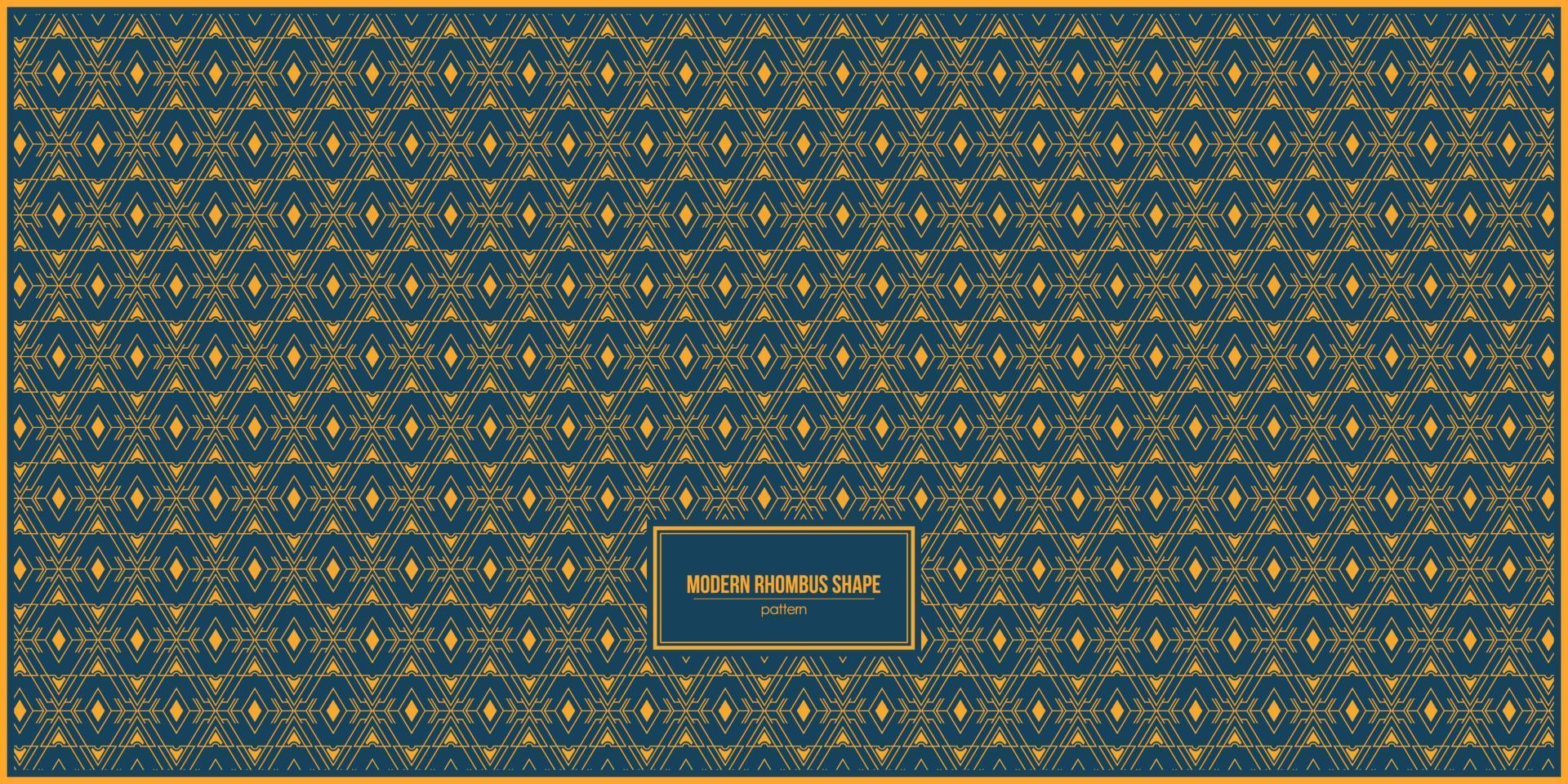The image is a horizontal rectangle adorned with a repeating geometric pattern in two-tone shades of teal blue and tan orange, though some describe the colors as dark blue and gold. Each design element consists of a smaller diamond at the center, encapsulated by a larger diamond of a contrasting color. This pattern is meticulously repeated across the surface, appearing around 200 times, creating a tapestry-like effect. Nestled within the bottom third of the image is a rectangular text box with the words "MODERN RHOMBUS SHAPE" prominently displayed in all caps. The intricate design and close arrangement of shapes give the appearance of a sophisticated wallpaper or gift wrap. Additionally, there's a gold line framing the entire rectangle, adding a finishing touch to this modern, artistic composition.